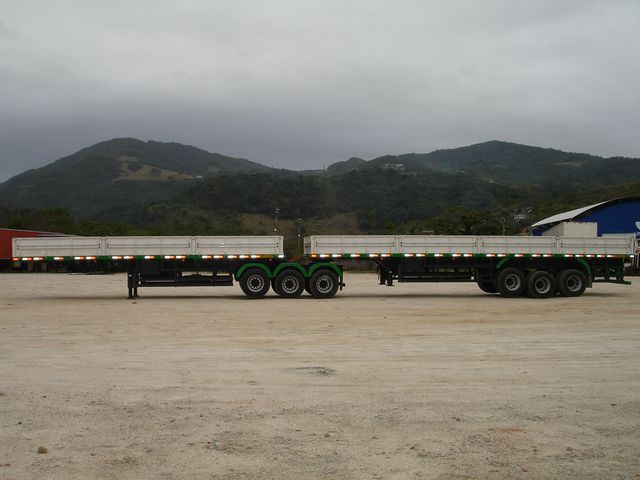The detailed photograph captures a scene set in a fog-covered outdoor environment. In the foreground, there is a long semi-truck trailer without its cab, appearing to be parked on a gravel-like surface. This trailer seems to be part of a truck's load-carrying section, with six wheels visible—three underneath the midsection and three at the end. The setting features another trailer positioned near it, also without its cab, suggesting they may be connected or side-by-side. This second trailer also shows a similar wheel arrangement. Behind these trailers, there are greenish, dark green, and brown mountain ranges, creating a striking backdrop. Amidst the mountains, there are patches of trees, and a building, described to be blue and white, is visible behind one of the trailers. The ground beneath the scene is described as light-colored dirt. Above, the sky merges with the fog, presenting a very light, faded blue shade with traces of white clouds, creating an almost surreal atmosphere with no distinct sight of the sun or clear sky.